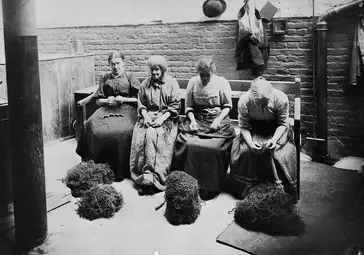This small, black-and-white photograph features four women seated on a single wooden bench against a brick wall. All four women are dressed in modest, long dresses appropriate for an older era. They each have their hands positioned in their laps, with one woman on the far right leaning forward and another in the middle appearing to work meticulously on something. In front of the women are four mounds that resemble either clumps of moss or mops, suggesting they might be involved in some sort of textile or craft work. The backdrop includes a stove pipe and some hanging garments, such as hats and jackets, which hints at an industrial or factory setting. The scene is quite sparse, emphasizing the utilitarian nature of their environment.